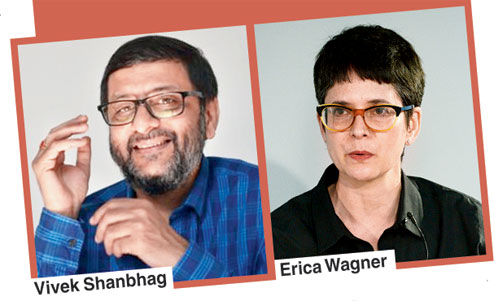In the photograph, there are two people standing side by side in what appears to be a portrait setting. On the left is a man named Vivek Shanbhag, identifiable by his slightly awkward smile and the gesture of his raised hand near his head, with one hand open. He has black hair and is dressed in a plaid shirt featuring shades of blue and navy. 

Next to him is a woman wearing a black button-down shirt with a collar. She has dark brown, almost black hair and is also sporting glasses, which have a mix of brown and black. Both individuals are wearing glasses, though his frames are predominantly black. 

The background showcases a light-colored wall, with a surrounding area painted in a peachy-orange to reddish hue, adding warmth to the portrait's setting. The details and attire of the subjects, combined with their expressions, contribute to a candid, intimate atmosphere captured in this well-composed photograph.